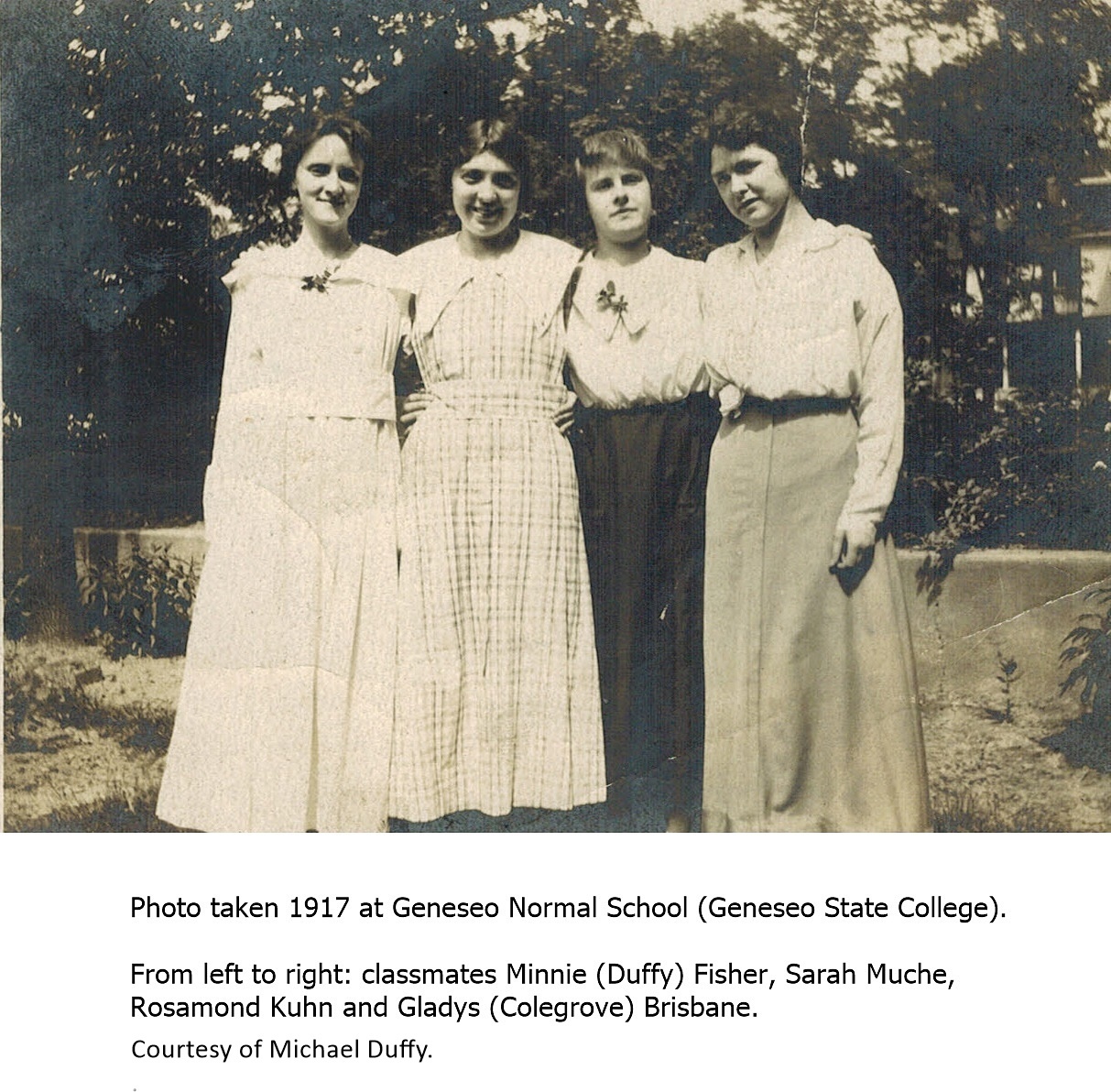This black-and-white photograph, taken in 1917 at Geneseo Normal School (now Geneseo State College), depicts four young women standing in front of a backdrop of trees and a concrete retaining wall. From left to right, the classmates are identified as Minnie Duffy Fisher, Sarah Mooch, Rosamund Kuhn, and Gladys Colgrove-Brisbane. All four women, donned in attire characteristic of the era with long skirts and blouses, are smiling at the camera. The first woman on the left is dressed in a white dress, the next in a white checked dress, followed by one in a white top paired with a black skirt, and finally, the woman on the right wears a white top with a lighter-colored skirt. They have short, dark hair and are adorned with brooches, reflecting the fashion of the time. This image, courtesy of Michael Duffy, captures a moment of camaraderie and elegance against the natural and architectural elements of their surroundings.